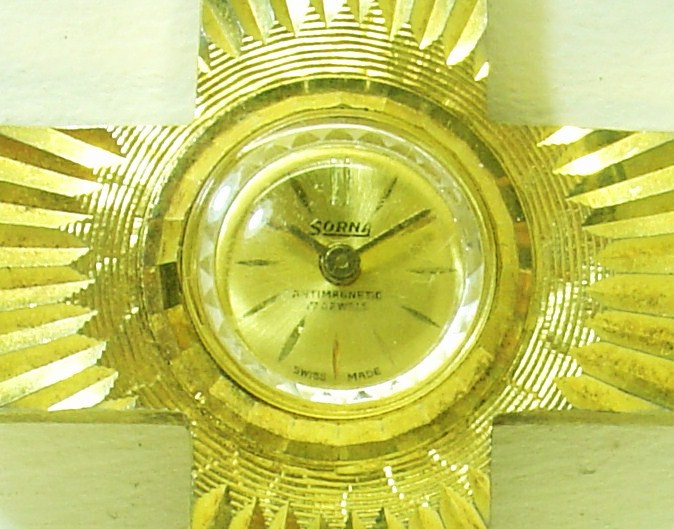The photograph features a strikingly yellow, gold-toned wall clock designed with a cross-shaped frame. At the intersection of the cross, a circular, glass-covered clock face is nestled, adorned with radiating, sun-like rays emanating from its center. The clock face features elongated dashes instead of numbers to mark the hours, and reads the time as 10:10. The brand name "SORNA," along with the inscriptions "anti-magnetic" and "Swiss made," are prominently displayed on the dial. The piece, set against an off-white or pale yellow backdrop, exudes an overall luxurious, ornate appearance, making it appear suitable for advertising. The clock’s frame may resemble a shell texture or a maple wood finish, enhancing its rich, extravagant aesthetic.